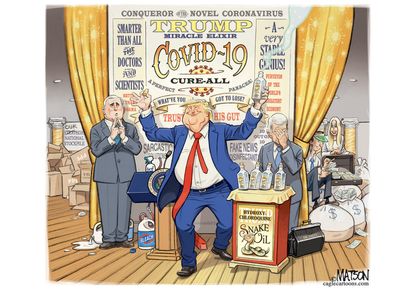The image is a highly detailed political cartoon signed by Mattson, depicting a satirical scene featuring former President Donald Trump. In the cartoon, Trump is portrayed in a cartoonish manner, wearing a blue suit, white shirt, and an exaggeratedly long red tie. His facial expressions are exaggerated to the point of novelty, and his tie comically wraps around his leg resembling a snake. Trump stands on a wooden stage holding a bottle of water in his left hand, with his arms outstretched.

To the left of Trump, a caricature of former Vice President Mike Pence is seen in a gray suit with a blue tie and short white hair, holding his hands together as if in prayer, sporting an unusual expression. To the right of Trump is a caricature of Dr. Anthony Fauci, depicted with a gray suit and his head in his hand, exuding distress.

In front of Trump is a podium labeled "snake oil," adorned with several bottles and topped with an illustration of a snake. The backdrop features large yellow curtains with a sign proclaiming "Trump Miracle Elixir, COVID-19 Cure-All," clearly mocking the promotion of dubious pandemic cures. Bags of money with dollar signs are strewn in the background, suggesting a lucrative scheme, further emphasizing the cartoon’s critique of exploiting the COVID-19 crisis. A bottle of bleach is also depicted behind Trump, adding another layer to the satire.